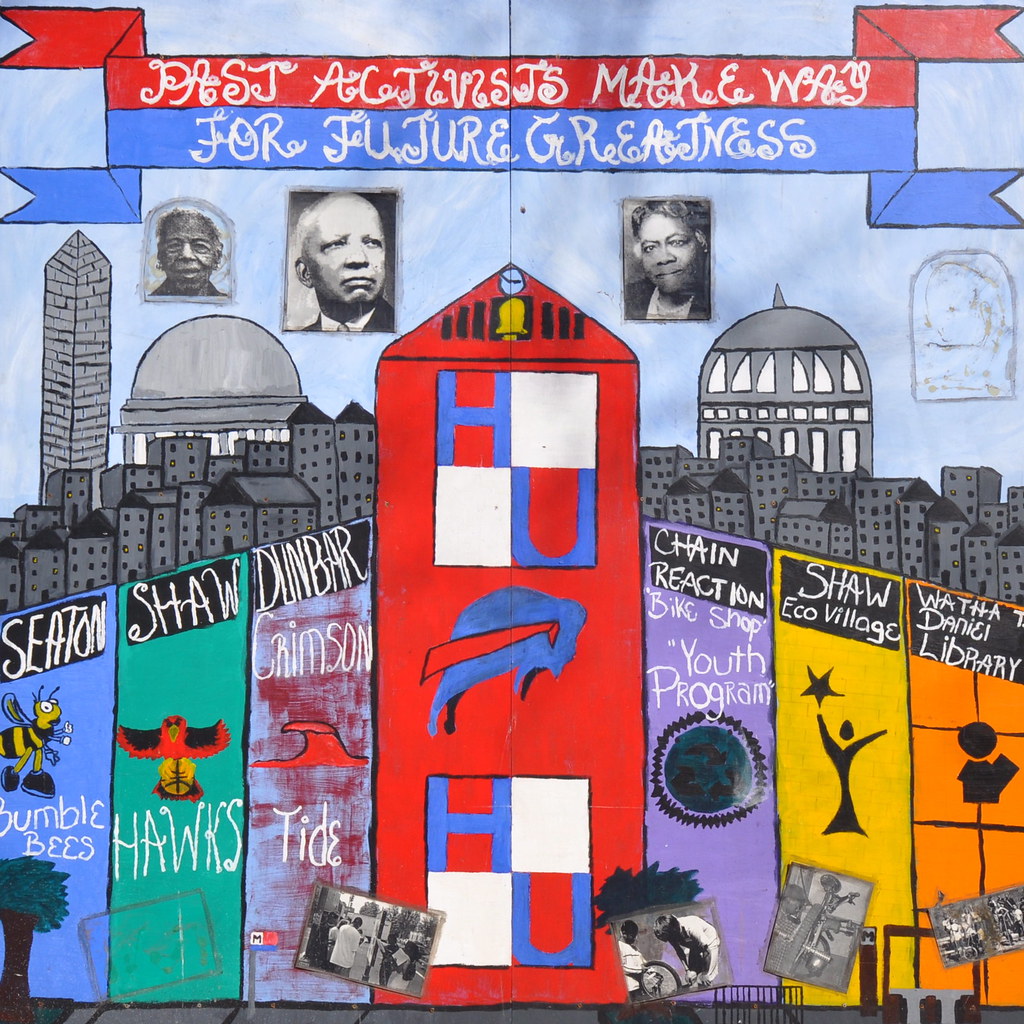The mural is a vibrant and colorful piece of street art that blends elements of cartoon and painted graphics, creating a lively scene. It features a city skyscraper background set against a series of sectioned-off stripes on a lower wall, each in distinct colors: blue, teal, light purple, red, yellow, and orange. Each stripe highlights different community and activist themes, with text names such as Seton Bumblebees, Shaw Hawks, Dunbar Crimson Tide, Chain Reaction Bike Shop Youth Program, Shaw Eco Village, and Watch Denon Library. Each section also contains corresponding paintings, including a bumblebee, a hawk, a tidal wave, a tree with a star on top, and a cartoon icon holding a book. 

At the top of the mural, a red and blue banner reads "Past Activists Make Way for Future Greatness," celebrating the legacy and contributions of African-American leaders. Among the graphics, there are black-and-white photographs of three African-Americans: two men and one woman, honoring their historical significance. Additional smaller black-and-white images appear at the bottom of the mural, though their details are less discernible. The mural collectively pays homage to past achievements while inspiring future generations with its dynamic imagery and community-centric themes.